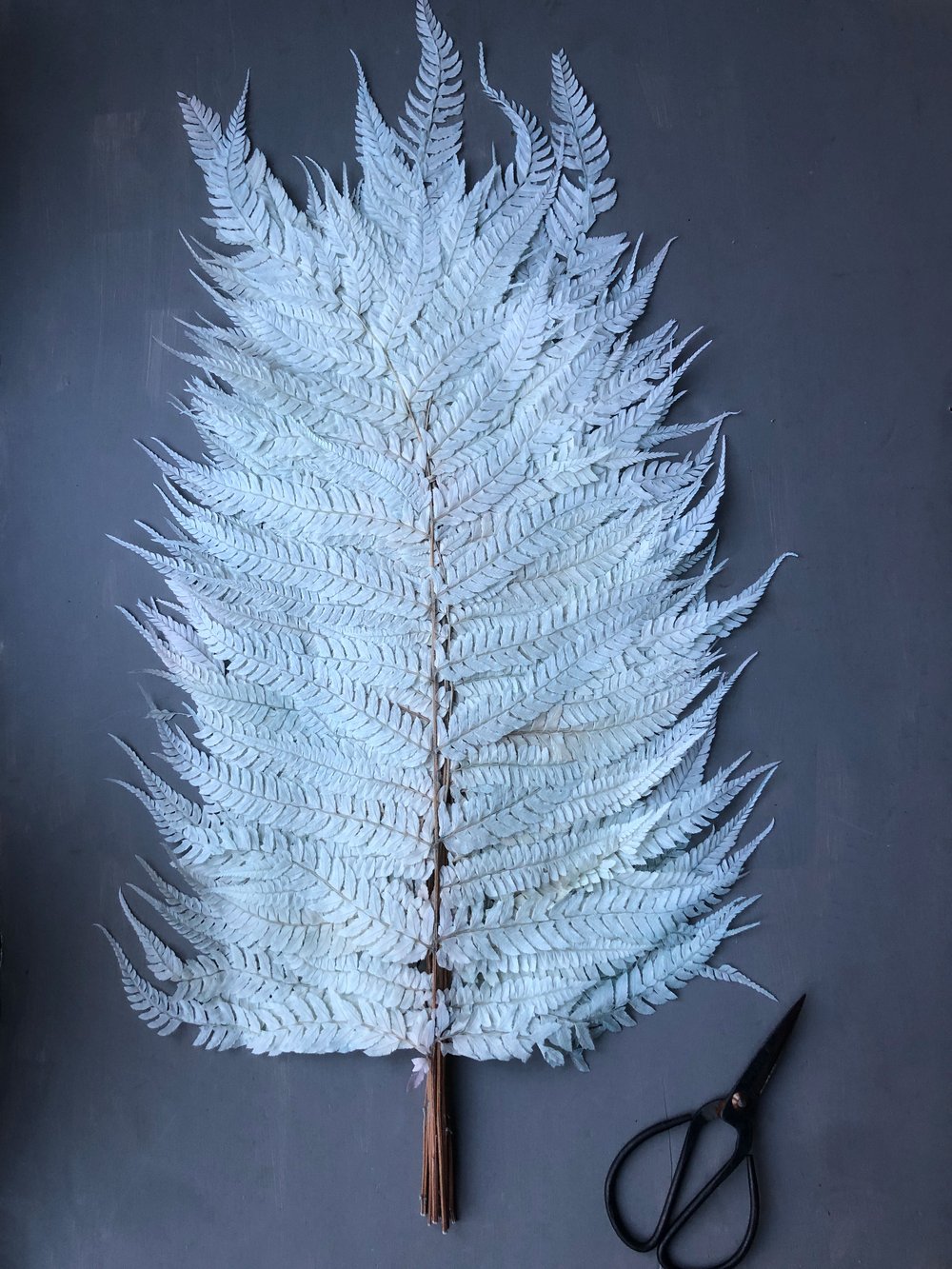The photograph captures an intricate handmade fan created from plant materials, displayed on a blue table. The background fades from a darker blue at the corners to a lighter blue towards the center, suggesting a gradient effect. The fan is composed of brown twigs at the base, which act as a handle, and white, thin, segmented leaves sprouting densely from both sides and slightly at the top, giving it a feathered appearance. The leaves are meticulously arranged without much space between them, creating a cohesive and dense structure resembling a fan or a miniature tree from afar. Near the bottom right corner of the image, a pair of black metal scissors with rusted areas around the central screw lies, indicating the craftsmanship involved in making the fan. The closed scissors, with their large oval handles and sharp blades, add a touch of practicality and context to the artistic scene.